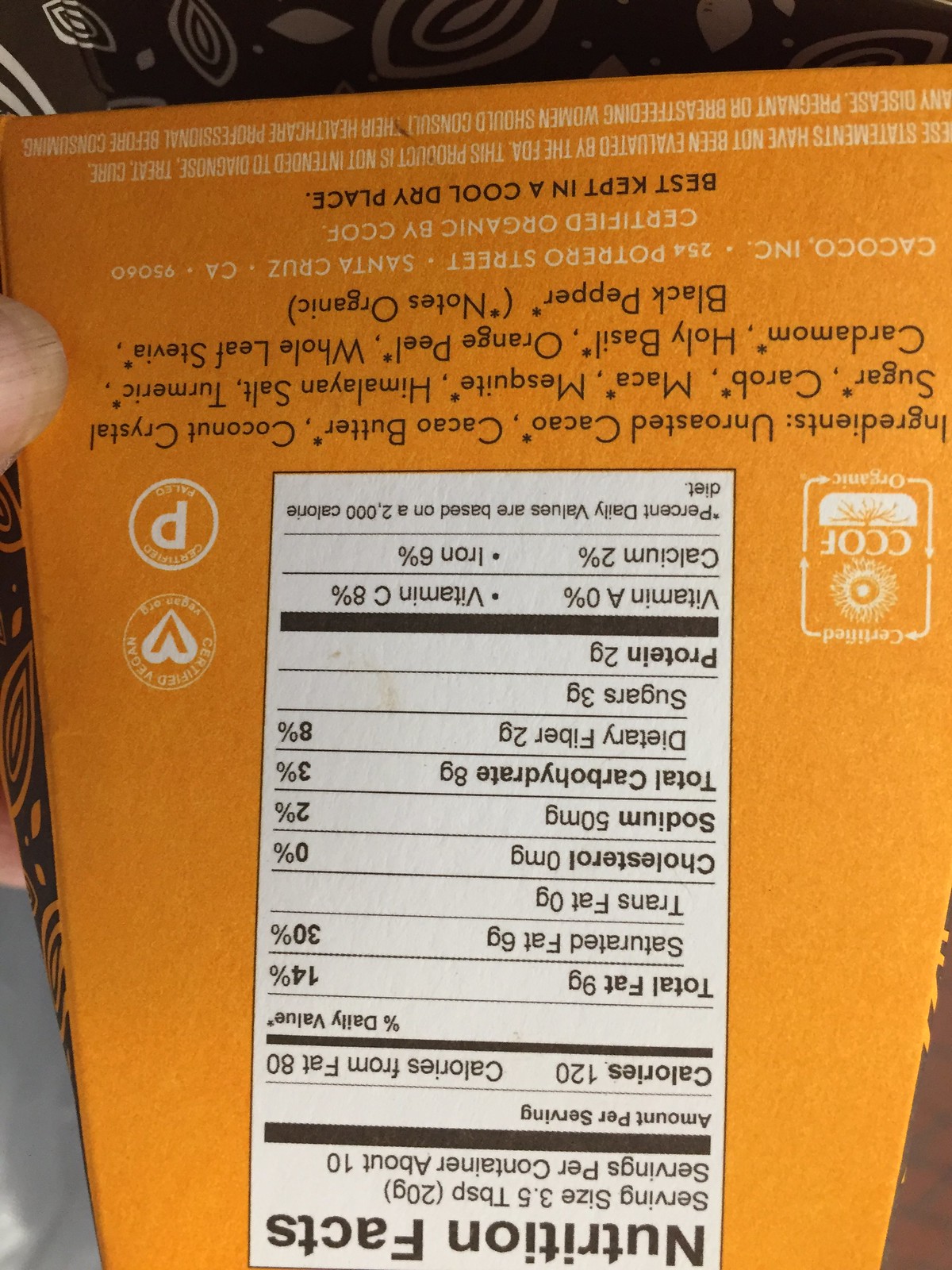The image features an upside-down photograph of an orange food package displaying its nutritional information. The packaging background is predominantly orange with black and white text. The nutritional facts box is visible from the bottom of the frame, with detailed information such as 120 calories, 9 grams of total fat, 6 grams of saturated fat, 0 trans fat, 0 cholesterol, 50 mg of sodium, 8 grams of total carbohydrates, 2 grams of dietary fiber, 3 grams of sugar, 2 grams of protein, 0% vitamin A, 2% calcium, 6% iron, and 8% vitamin C per serving. Additionally, the packaging is certified organic by CCOF, certified vegan, and certified paleo. The ingredients include cacao, holy basil, black pepper, and orange peel, suggesting a chocolate product. The text also indicates the product is best kept in a cool place. There is a noticeable finger holding the box from the left side, emphasizing the upside-down orientation of the image.